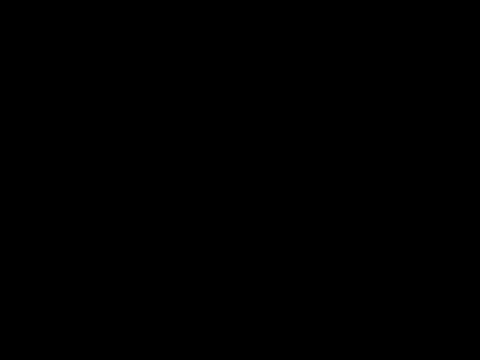The image displays a completely black rectangle that stretches across its entire surface, enveloping the viewer in a deep, richly black expanse with a slight reddish undertone. There are no highlights, shadows, lowlights, or discernible details visible anywhere within the frame. The edges, corners, and bottom are indistinguishable from one another due to the uniformity of the blackness. The entirety of the image is devoid of objects, text, and any form of distinguishing features, remaining an unbroken field of pure black. This stark, featureless blackness elicits the notion of an abstract painting, yet it emerges with a striking simplicity, emphasizing its unremarkable and undisturbed nature.